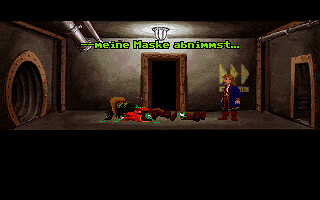In a dimly lit video game setting, the image portrays a grey, industrial room with metallic features. The walls are entirely grey, and the doorways are fashioned from a copper-like metal, reinforced with rivets giving them a sturdy appearance. On the left side of the room, a circular tunnel-like doorway is visible, accented with multiple smaller circles. The room's corners are fortified with the same copper metal, adding to the industrial aesthetic. A prominent silver pipe runs along the upper portion of the room, and at the very center of the ceiling, a light fixture casts an ambient glow over the space.

To the far right, another doorway made of copper and metal stands. At the back of the room, three yellow arrows are pointing to the right, directing towards a central doorway. On the floor, there is a red coat and a brown hat, hinting at perhaps a previous or ongoing presence. To the right of these items, a blue-clad person with brown hair and brown shoes stands, adding a human element to the otherwise mechanical environment.